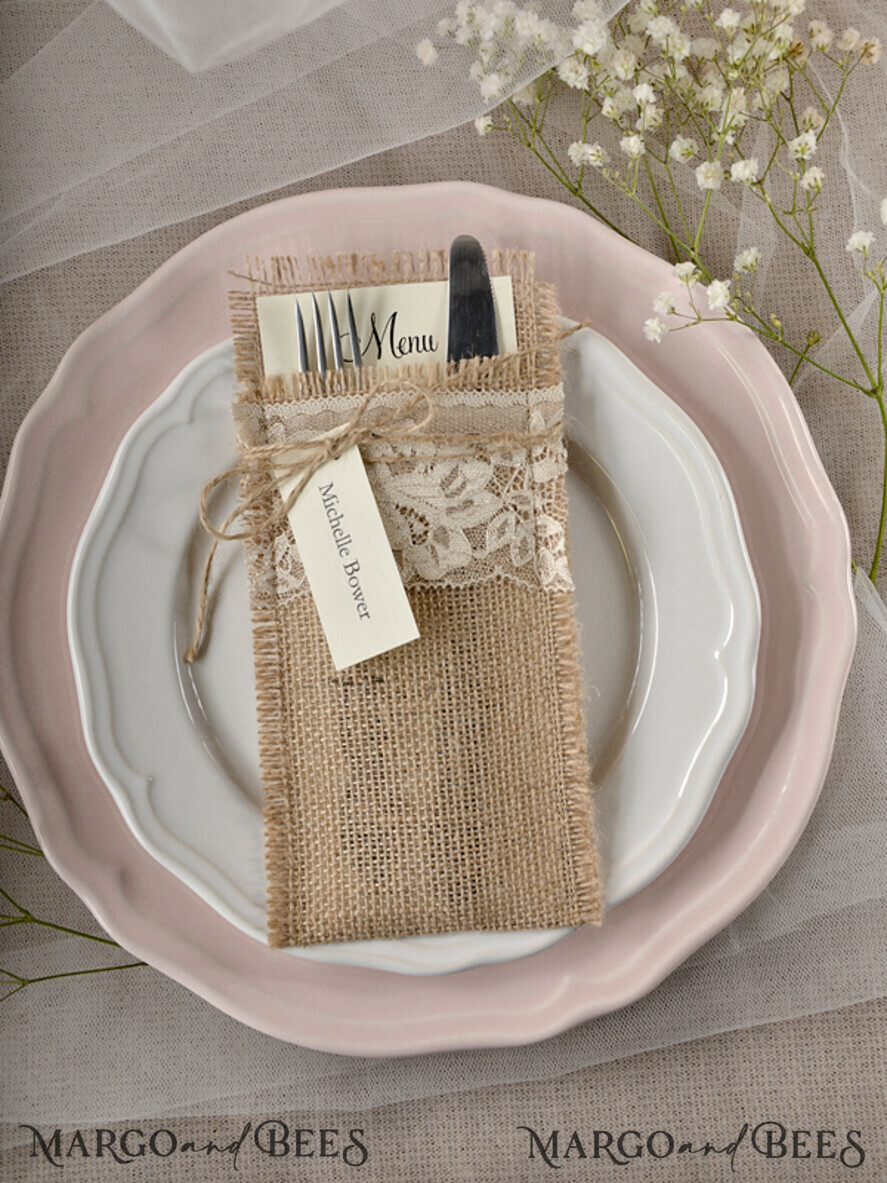The image depicts an elegantly arranged place setting, likely for a wedding. At the center, a burlap pouch with a lace strip wrapped around it is tied with twine, creating a charming pocket that holds a metal fork and knife, alongside a menu. A tag reading "Michelle Bauer" is affixed to the twine. This pouch is placed on a pristine white plate, which itself rests on a light pink charger plate. The entire arrangement sits on a silky white tablecloth that evokes the texture of a wedding veil. In the upper right corner, delicate sprigs of baby's breath with white flowers add a natural touch. The bottom left and right corners of the image carry a watermark with the text "Margot and Bees" in black.